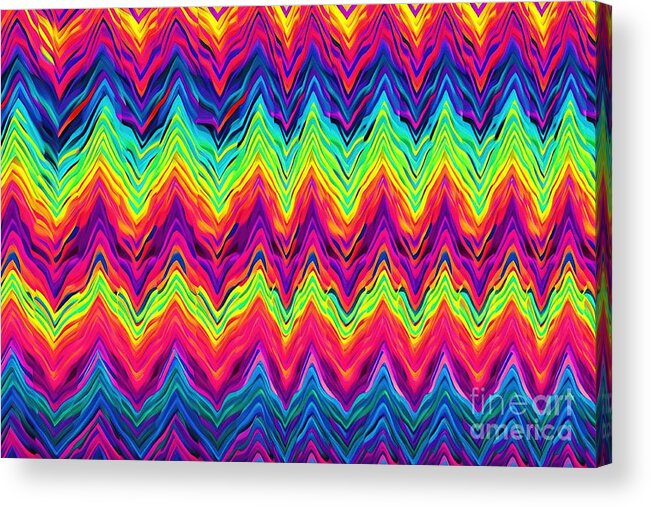This image is of a painting hanging on a wall without a frame, though there is a little visible edge of the canvas on the right side. The painting is likely oil on canvas and measures slightly over an inch in thickness. In the lower right corner, there's a faint, white watermark reading, “Fine Art America.” The artwork features a vibrant and modern rainbow-colored pattern composed of alternating up-and-down zigzag lines. These lines, resembling those you might see on a heart monitor, are arranged in sequences that start with purples in the center and transition outward into reds, oranges, yellows, greens, blues, and back to reddish tones. This highly colorful piece includes layers of these lines placed atop one another, creating an intricate and lively visual effect. The variety of colors includes bright yellows, pinks, aquas, blues, dark blues, and purples, forming a mesmerizing, repetitive pattern across the canvas.